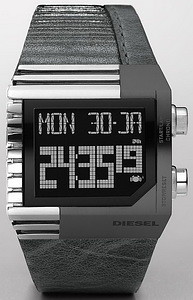This black and white digital wristwatch features a rectangular face with a detailed display. On the right side of the face, there are two knobs used for adjusting the date and time settings. The left edge of the watch face is adorned with silver ribbing, adding a touch of contrast to the overall design. The watch strap is a darker gray color, with visible stitching along the right side for added durability and style. The Diesel brand name is prominently displayed on the bottom right corner of the watch face. The digital display denotes the day as "Mon" for Monday, the date as "30-JAN" for January 30th, and the time as "24:35:19" seconds. This timepiece combines functional digital technology with a sleek and modern aesthetic.